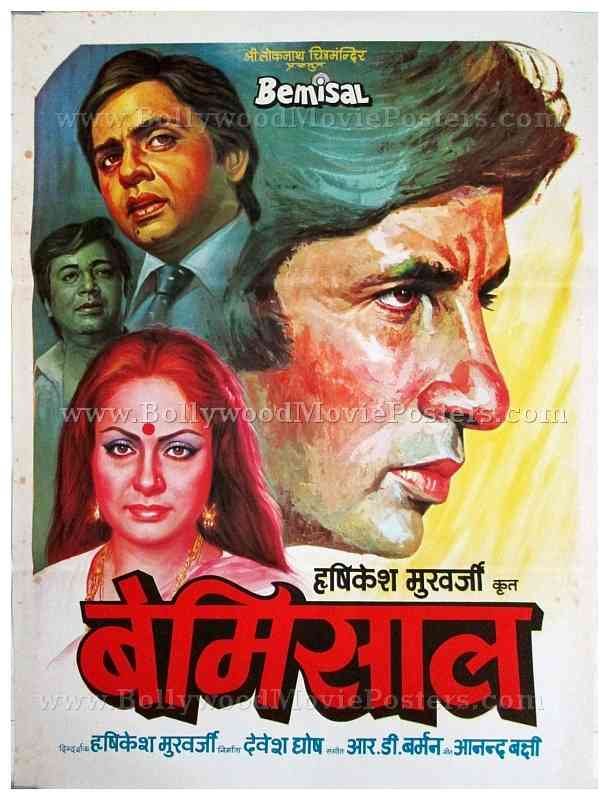The image is a scan of a Bollywood movie poster with transparent white text watermarks reading "Bollywood Movie Posters" and "www.BollywoodMoviesPoster.com." The poster is hand-painted and features a collection of human faces. Dominating the right side is a large, side-view face, while the left side displays three smaller faces stacked vertically. The topmost face is a man wearing a white T-shirt and black tie, the middle face is another man, and the bottom face is a woman dressed in a white dress and pink sari. The background shifts from blue at the top left to yellow at the bottom right, with a white section at the bottom. The title "BEMISAL" is prominently displayed at the top in white letters, while additional text in Hindi, including the film's name and actors' names, appears at the bottom in red and black.